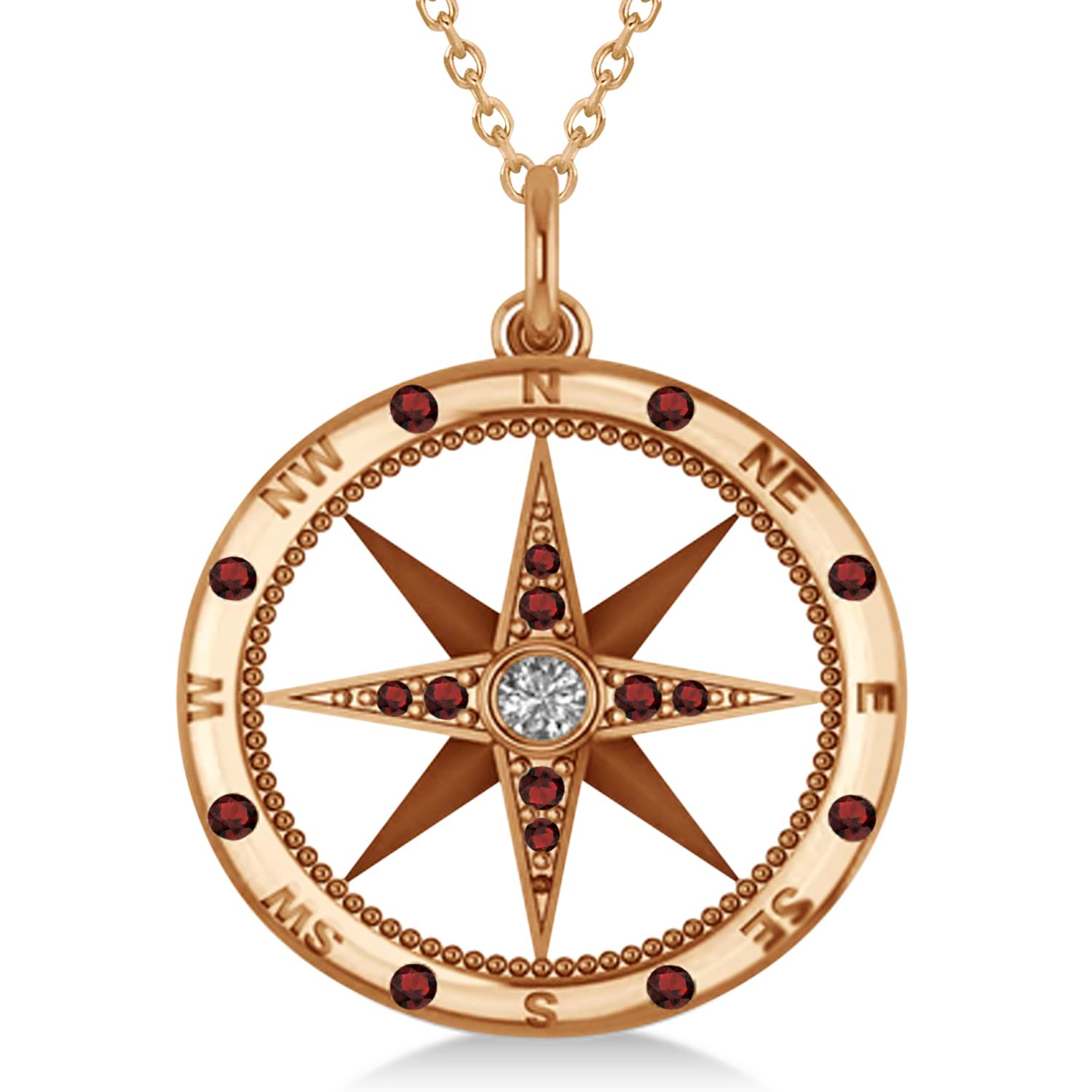The image features a gold necklace with a pendant designed to resemble a compass. The necklace has a short gold chain, visible at the top center, that curves downwards about an inch before looping back up. The pendant itself is a round gold medallion, slightly lighter in the central area. 

Encircling the medallion are raised directional markers: North, Northeast, East, Southeast, South, Southwest, West, and Northwest, each interspersed with small red rubies. The center of the pendant showcases a star with eight points: the back four points are plain brown, while the front four are gold and adorned with two rubies each. A small diamond is set at the very heart of the star. The pendant casts a slight shadow on the plain white background, accentuating its intricate details and the richness of its colors.